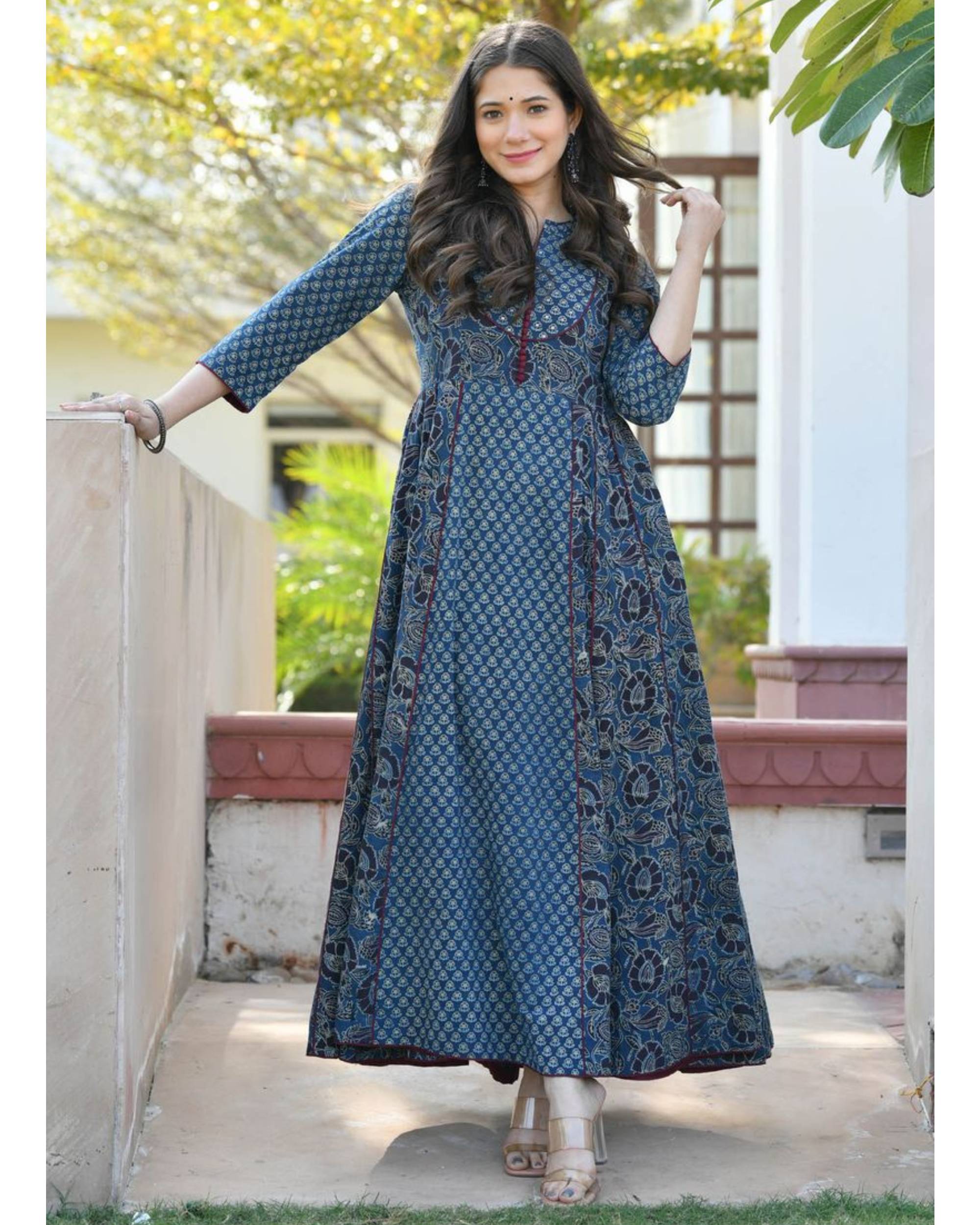In this vibrant outdoor portrait, a young Indian woman stands gracefully in front of a white house with brown trim, framed by lush trees and leaves in the background. She is dressed in an intricately patterned blue dress, featuring multiple shades that extend down to her beige high-heeled shoes. The dress has long sleeves and covers her entire body, reaching down to her feet. Her fingernails are painted a shade of blue similar to her dress, and she sports a silver bracelet on her right arm. Her dark, wavy hair cascades down as she holds a strand with her left hand, while her right hand rests elegantly on a nearby wall. She adorns a traditional jewel or marking on her forehead, which complements her radiant smile. The bright, sunny setting enhances the warmth and richness of the scene, capturing the essence of a serene and beautiful moment.